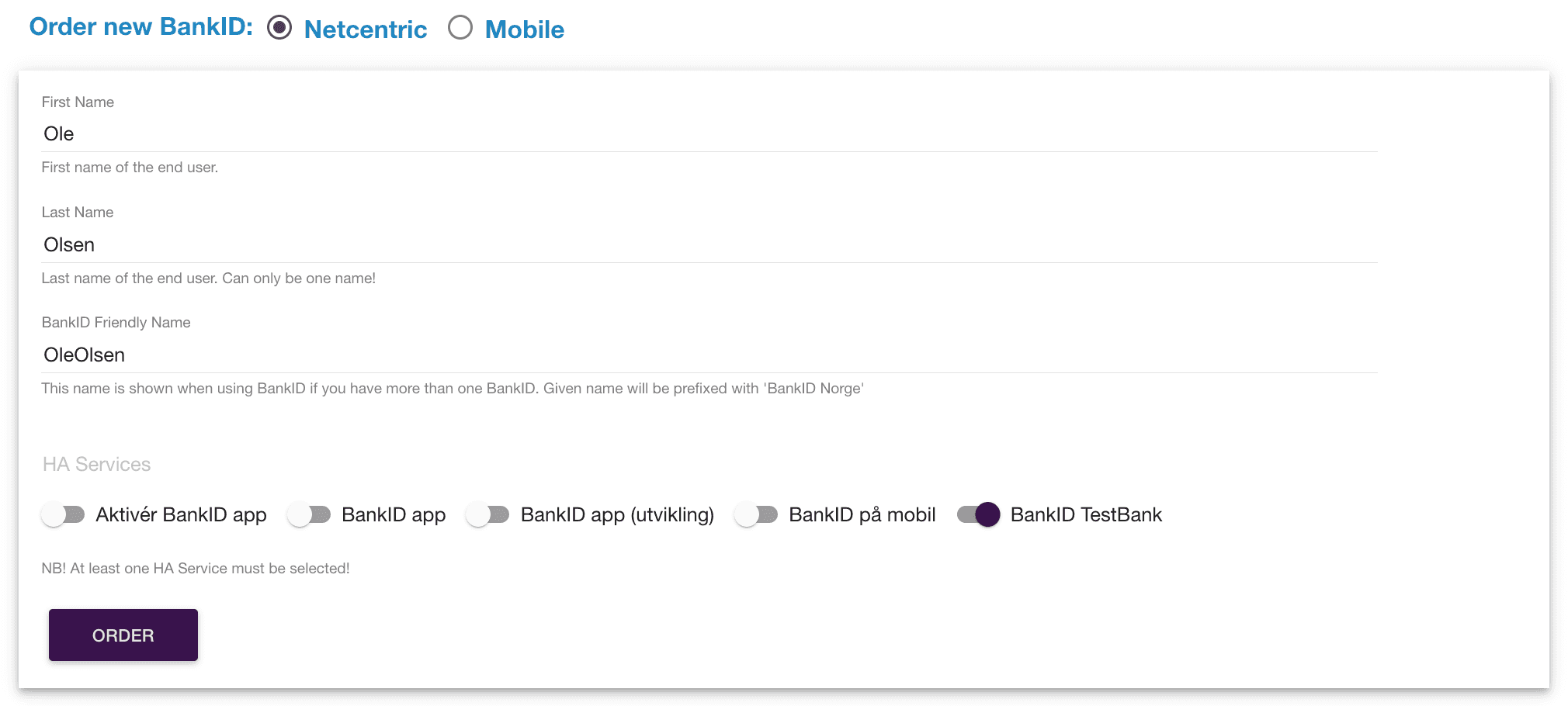The image depicts a web interface for ordering a new Bank ID. At the top, there are two options presented as radio buttons: "Net Centric" which is selected, and "Mobile" which is not. 

Below these options, there are input fields for the user's name. The fields display "Oli" as the first name and "Olsen" as the last name, with a note that this is the only permissible last name for the end user. Additionally, "Oli Olsen" is designated as the "Friendly Name" for the Bank ID, indicating that this name will be displayed when the user utilizes their Bank ID. If the user has multiple Bank IDs, the name will be prefixed with the Bank ID number in orange.

Further down, a section titled "HA Services" lists several buttons, some of which are toggled on or off:
- "Activa Bank ID App" (Status: Off)
- "Bank ID App UTVICLIN" (Status: Off)
- "Bank ID PA Mobile" (Status: Off)
- "Bank ID Test Bank" (Status: On)

A cautionary note below these buttons states, "N.B. N.B., at least one HA service must be selected." 

At the bottom of the interface, there is a dark purple "Order" button with white text, which the user can click to finalize their Bank ID order.